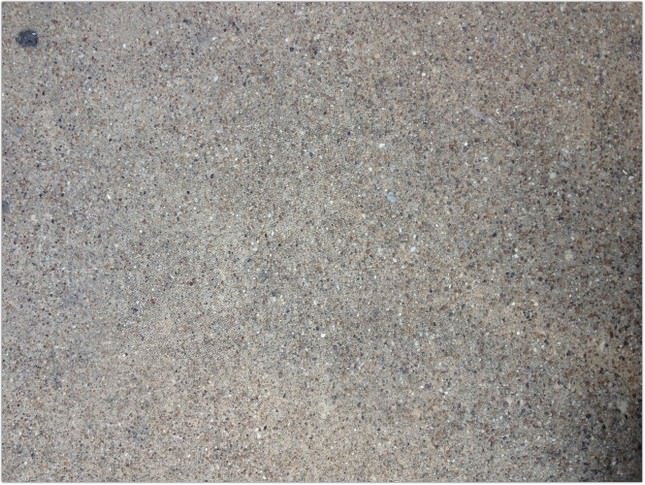The image showcases a piece of grey flooring, likely composed of smoothed-out concrete. To the left side of the frame is a small, greyish circle, adding an element of interest to the scene. Scattered across the surface are specks of varying shades, including grey, white, dark grey, and light grey, creating a textured and speckled appearance. The lighter shades add depth while avoiding a stark white contrast. In the top left corner, the grey darkens noticeably, possibly due to shadow, which gives a gradient effect culminating in a notably darker region on the bottom right side. This interplay of light and shadow across the grey tones enhances the visual complexity of the flooring.